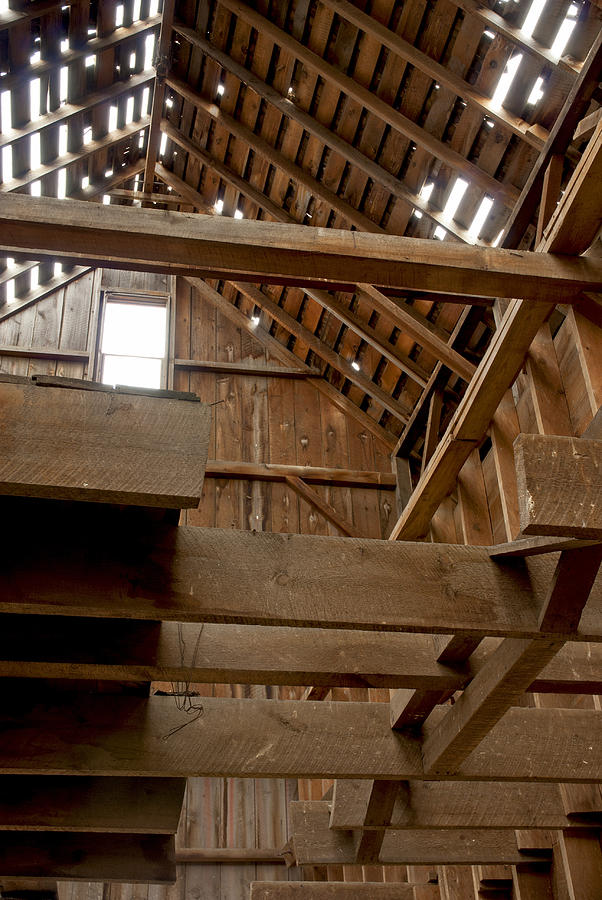This indoor color photograph captures the dilapidated interior of a wooden barn, taken from the ground level looking up towards the roof. The ceiling and floorboards of the second level are partially missing, revealing aged yet structurally sound wooden rafters and beams of various shades, primarily light to medium brown. The unfinished roof exposes slats with missing sheeting, allowing sunlight to filter in, accentuating the texture of the weathered wood. A beam spans horizontally across the upper third of the image, intersecting with other beams that run the length of the roof and connect at angles, suggesting potential walkways. A gable end window at the back of the barn allows additional light to penetrate the space, casting an aura of neglect and rustic charm. Despite its disrepair, with pieces of wood missing and visible holes looking out into the sky, the barn stands resilient, hinting at a past utility and the passage of time.